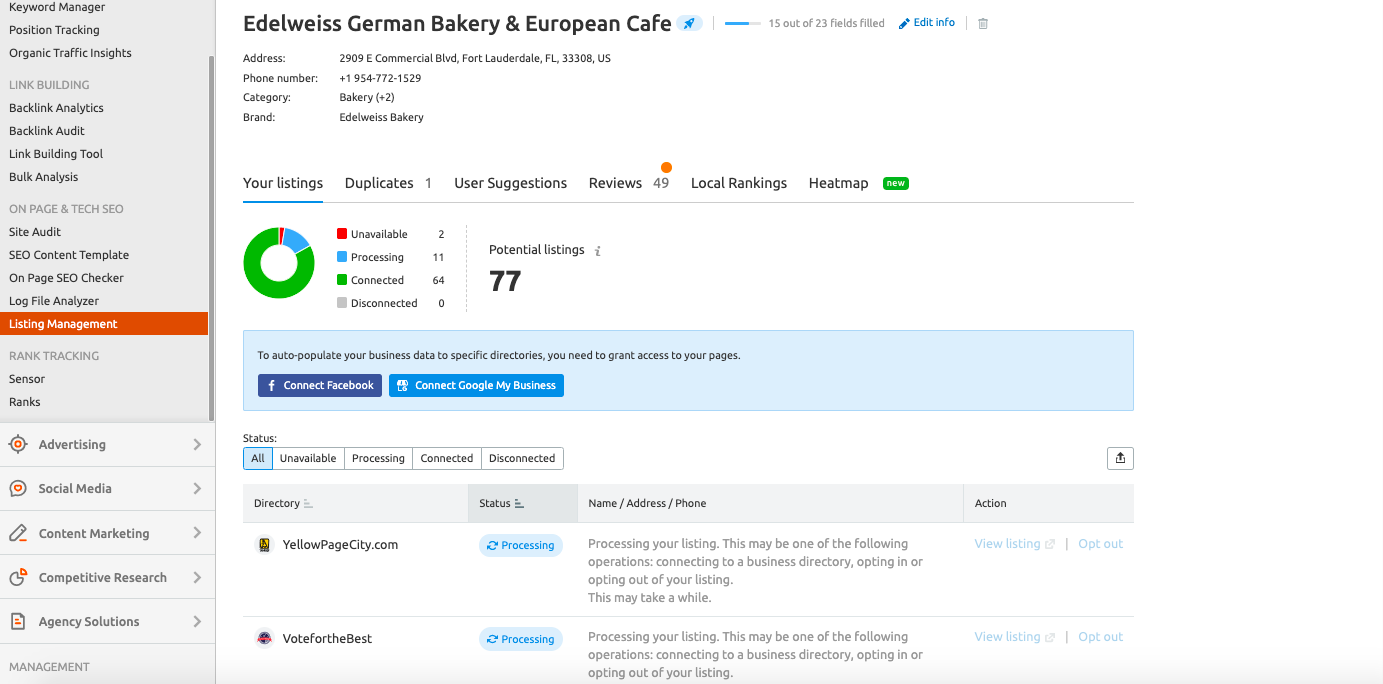In the screen capture, the interface is dominated by a light gray vertical menu on the left, occupying approximately a quarter of the total display. The remaining three-quarters of the screen, located to the right, features a white background that showcases dashboard information. 

The left side menu is organized with various options in black font, including:

- Keyword Manager
- Position Tracking
- Organic Traffic Insights
- Link Building (and its subcategories such as Backlink Analytics, Backlink Audit, and Link Building Tool)
- Bulk Analysis
- On-Page and Tech SEO (which further includes Site Audit, SEO Content Template, On-Page SEO Checker, and Log File Analyzer)
  
A section highlighted in orange, featuring white font, stands out with options like:
- Listing Management
- Rank Tracking
- Sensor Ranks

Additionally, there are expandable menu items that are currently not opened, such as:
- Advertising
- Social Media
- Content Marketing
- Competitive Research
- Agency Solutions

On the right-hand side, under the "Listing Management" section, detailed information is displayed for a specific business named "Heidel Weiss German Bakery and European Café." The details include the business's address, phone number, and category, noting the brand as "Heidel Weiss Bakery." There are also options available for managing the listing, checking duplicates, and other relevant tasks.